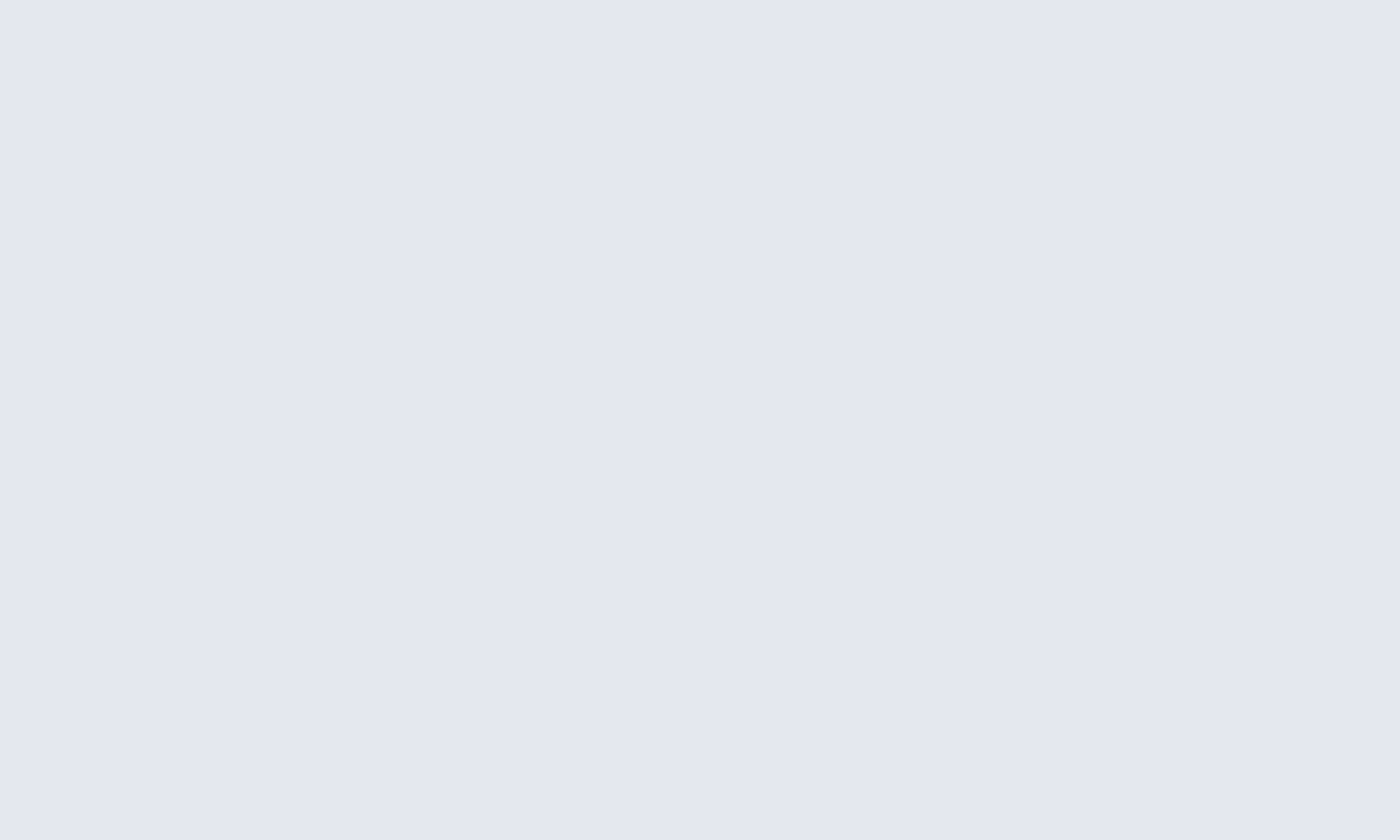A large, light gray rectangular box occupies the entire area, devoid of any text or images. Measuring approximately eight inches horizontally and seven inches vertically, this box is completely empty, providing a blank canvas in a subtle shade of light gray.